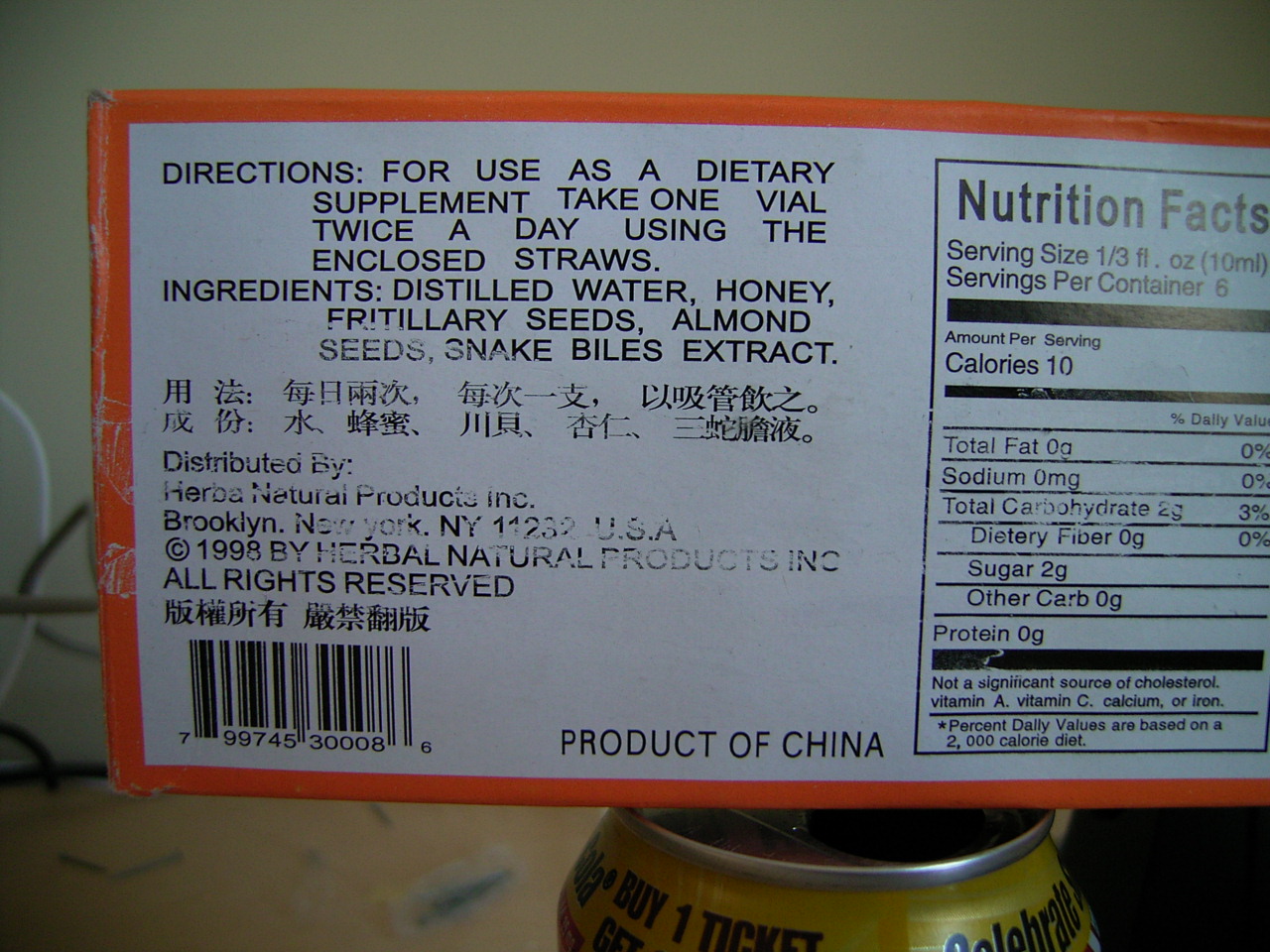Displayed in the image is the backside of an Asian product box, resting precariously atop a soda can or a similarly sized can. The box features a distinctive orange border framing a white interior adorned with black text. This text includes both the nutrition facts and detailed instructions for use. According to the directions, the product should be consumed twice daily, one vial per serving, with the help of an enclosed straw.

The ingredient list is prominently displayed and comprises distilled water, honey, fritillary seeds, almond seeds, and snake vials extract, the latter of which might raise ethical concerns due to its source. Beneath these details, some text in an Asian script is visible, followed by information stating that the product is distributed by Herb's Natural Products, based in Brooklyn, New York. Additionally, it mentions that the product is manufactured in China.

A barcode is situated to the left side of the box, while the right side presents the nutrition facts. The serving size is listed as 1/3 fluid ounces, with each container holding six servings. Notably, each serving contains 10 calories, with carbohydrate content at 2 grams, sugar at 2 grams, and zero fats, sodium, or proteins.

In the background of the image, a jumble of wires can be vaguely seen, and the can atop which the box is balanced rests on what appears to be a tablecloth, adding to the everyday setting of the scene.